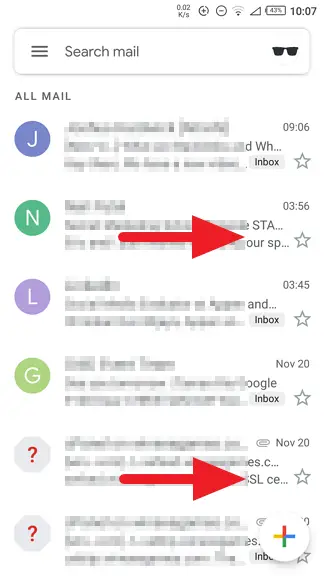The image is a screenshot from a phone, capturing various on-screen elements. The upper left-hand corner is empty, leading towards the middle where it displays "0.02 K/s." Adjacent to this are two unidentifiable circular icons. The Wi-Fi icon shows two bands, and next to it is a triangular symbol. The battery icon indicates a 47% charge. The time reads 10:07.

Below these indicators, there is a gray-outlined rectangle, white inside, containing three vertical bars stacked on top of each other, accompanied by the text "Search mail." To the right is an icon of black sunglasses. Outside this box, the label "All Mail" is displayed, along with six pieces of mail.

Each mail item has a colored dot with a letter inside: the first has a purple dot with a white "J," the second a green dot with a white "N," the third a lavender dot with a white "L," and the fourth a lime green dot with a white "G." Additionally, there are two large red arrows pointing to the right on the second and fifth mail items.